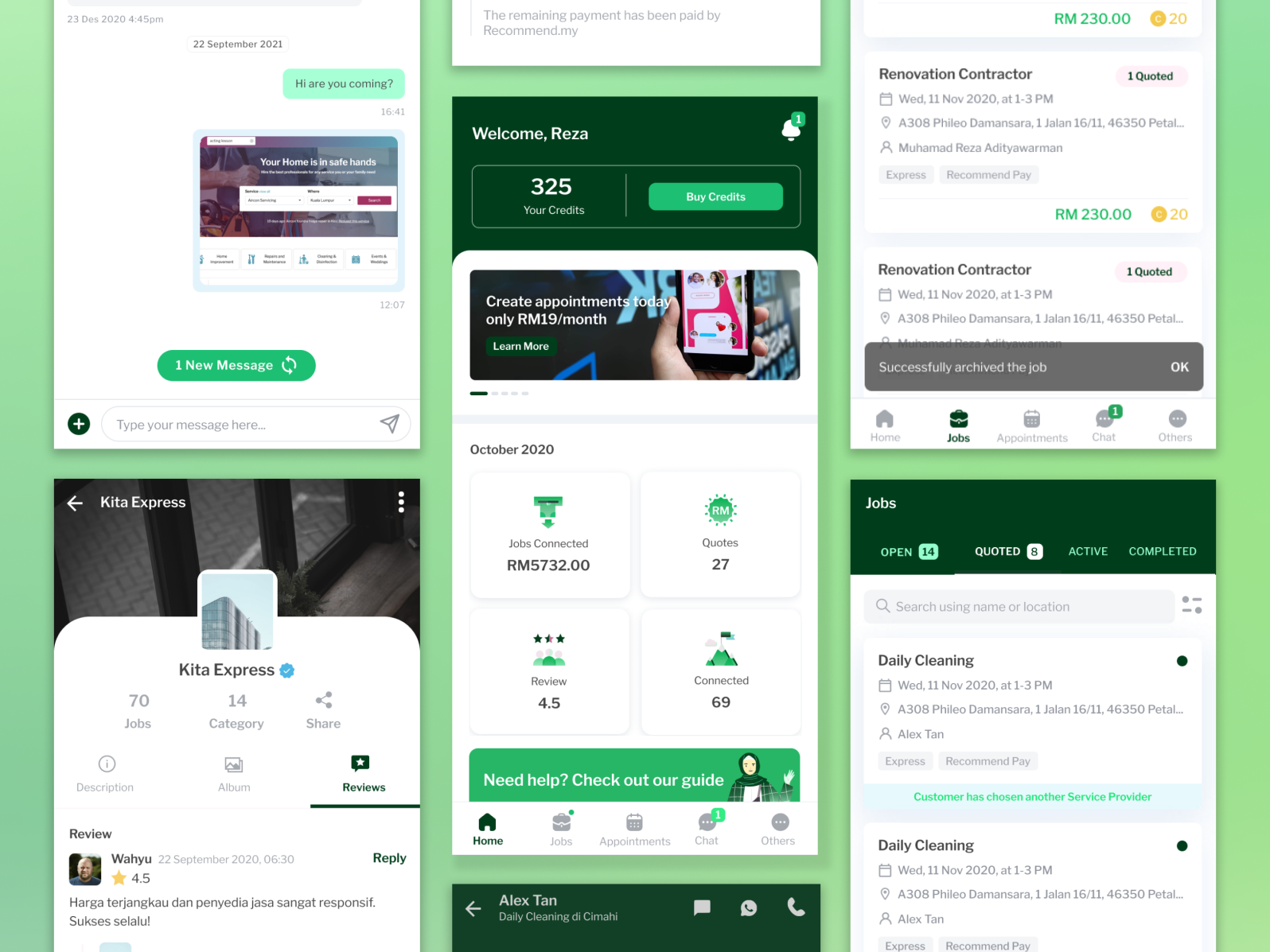**Category: Websites**

The image features a composite of various website elements and messages, seemingly strung together in a collage-like manner. Here's a detailed breakdown:

- **Top Left Section:**
  - A snippet showing a timestamp "23 December 2020, 4:55 p.m."
  - A message asking, "Hi, are you coming?"
  - Another snippet reassuring, "Your home is in safe hands."
  - An indicator displaying "one new message."

- **Middle Left Section:**
  - A header titled "Kita Express" featuring a message in a non-English language.
  - A text block mentioning "70 jobs category 14 share."

- **Center Panel:**
  - A notice stating, "Remaining payment has been paid by recommend my Welcome Risa 325."
  - A prompt offering, "Create appointment today only RM 19 a month learn more."
  - Tabs and categories listed as "October 2020 jobs contact jobs connected quotes review and Connected need help Check out our guide."

- **Bottom Row:**
  - Mention of "renovation character."
  - Information about "jobs daily cleaning."
  - A date and time reference: "11 November 2021 to 3."

The elements are haphazardly arranged, creating a chaotic yet intriguing visual representation of interconnected website pieces and messages, highlighting various features and notifications in a fragmented manner.